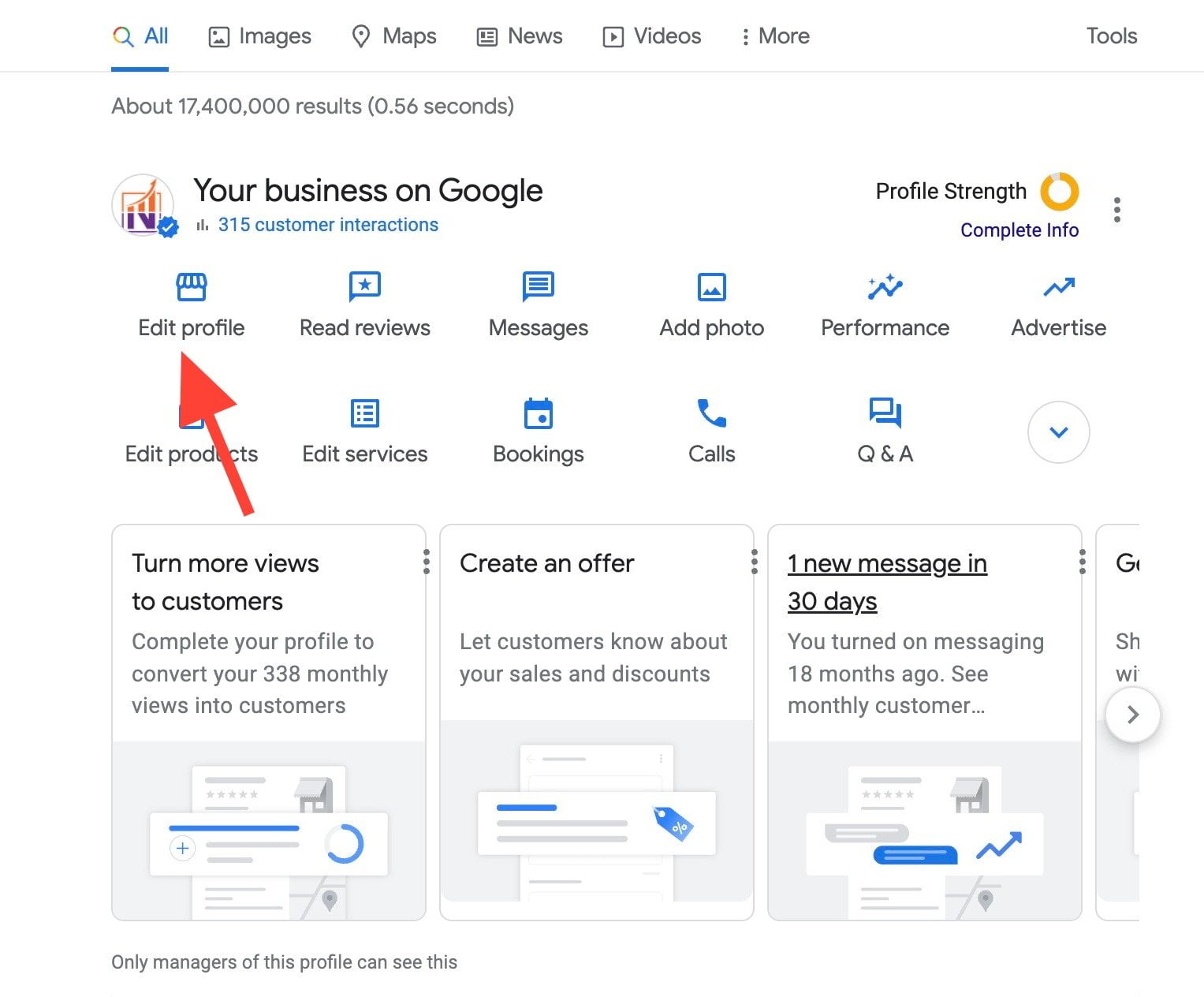The image displays a Google search results page, prominently featuring the following categories: Images, Maps, News, Videos. The search yields approximately 17,400,000 results in 0.56 seconds. 

In the foreground, a business profile interface is shown with various actionable insights and tools for optimizing the business's presence on Google. Key metrics include 315 customer interactions and profile strength, with prompts to complete info, edit profile, read reviews, and manage messages. 

Additional sections emphasize adding photos, monitoring performance, advertising, and editing product and service information. The business is encouraged to leverage features like bookings, calls, and questions and answers to increase customer engagement.

A highlighted message advises the business to "turn more views to customers" by completing their profile to convert their 338 monthly views into actual customers.

The interface suggests creating offers to inform customers about sales and discounts. It also notes that there has been one new message in the last 30 days and mentions that messaging was activated 18 months ago. Monthly customer insights are also accessible.